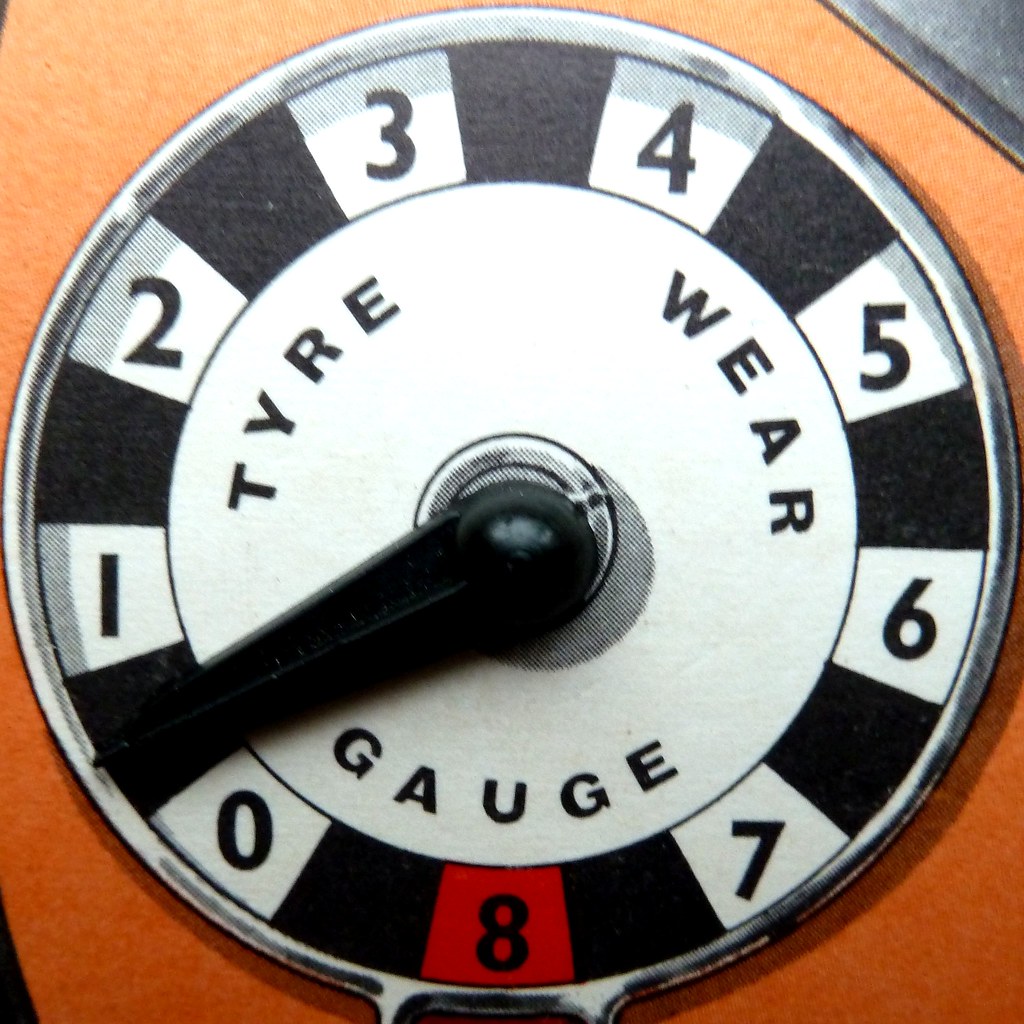This detailed square photograph showcases a black and white tire wear gauge with a textured, orange background, which spans all corners except the top right that has a small black spot. The gauge, centered in the image and encased in a silver frame, features numbers from 0 to 8 distributed around its circular edge, with each number positioned against alternating black and white squares. Notably, the number 8 at the bottom is highlighted with a red square, signaling a critical level. The gauge face prominently displays the words "Tire Wear Gauge" in black text against a white background. The gauge’s black dial points to the empty black square between the 0 and 1 markers.